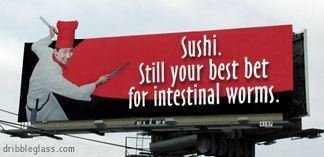This is a small, horizontal, rectangular photograph of a billboard set against a hazy sky. The billboard features a striking design composed of red, white, and black colors. On the left side, taking up about a third of the billboard, is a black section shaped like the letter "C" that extends into the lower right corner. 

Prominently featured on the left side is an image of a smiling chef wearing a tall red chef's hat, a white coat, and white pants. The chef is positioned with his body facing the right edge of the billboard while his head is turned slightly towards the viewer. He is holding a knife in his right hand and another utensil in his left hand.

The billboard's main background color is red, and it displays bold white text across the red area. At the top, the text reads "Sushi" in capitalized letters. Below that, in smaller text, it says "Steal your best bet," and at the bottom, it concludes with "for intestinal worms." The text is clean and clear, making an unusual and attention-grabbing statement.

In the lower left corner of the image, outside the billboard, is the URL "dribbleglass.com" in lowercase letters. The billboard is supported by a visible black framework, and some supporting wires can be seen extending from the lower left to the lower center.